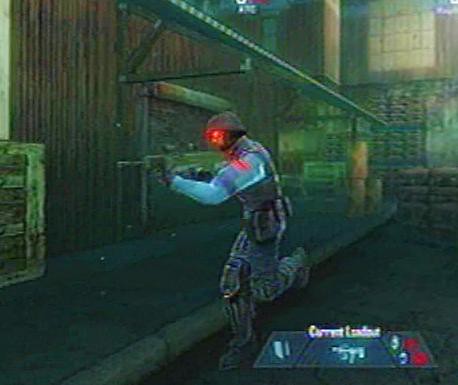The image is a screenshot from a video game, depicting a hazy, dimly-lit scene dominated by dark and light green tones. The environment resembles an industrial warehouse setting, with steel pipes running across the ceiling and stacked pallets or boxes visible towards the center-right of the ground. In the bottom right corner of the image, there is a rectangular interface element with unreadable white text that likely indicates an in-game status or instruction—potentially reading "CURRENT SOMETHING."

A central figure, presumably a soldier or military personnel, is captured mid-motion, running from the top right to the lower left of the frame. He is clad in a dark-colored uniform, including black pants, a black vest, a helmet, and a distinctive blue sleeve and armband on his left arm. His eyes ominously glow red through the visor of his helmet, and there is a red patch on his upper shoulder that might suggest he has been shot. The soldier is armed with a rifle or machine gun, poised and ready to fire. The overall poor image quality and significant blur contribute to the mysterious and intense atmosphere of this moment.